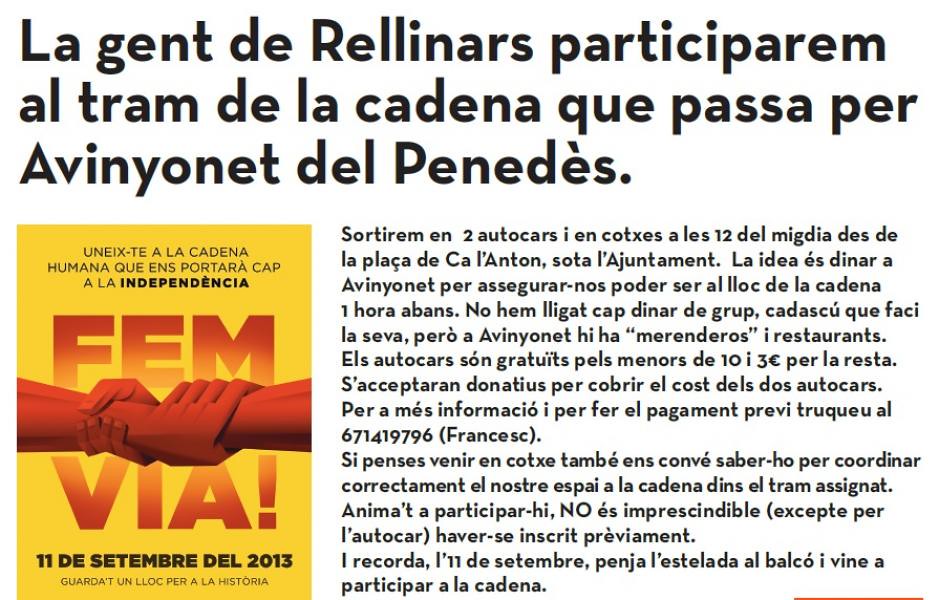The image displays a multi-colored print piece predominantly in Spanish, serving as an advertisement or poster for an event dated September 11, 2013. The background is largely black and white text, with a prominent headline in a larger, darker black font, above two paragraphs of additional text. Positioned in the lower left quadrant of the image is a striking yellow box containing black and red text. In the middle of this yellow box, two red arms and hands grasp each other's wrists, reminiscent of a rescue attempt. Above this visual, the red text reads "FEM," while below it, the text reads "VIA!" At the bottom of the yellow box, the date is presented as "11-D-September-Del-2013." The top of the poster features a headline in black text: "UNEX TE ALA GADENA HUMANA KE ENS PORTARA CAP ALA INDEPENCIA," indicating a call for unity towards independence.